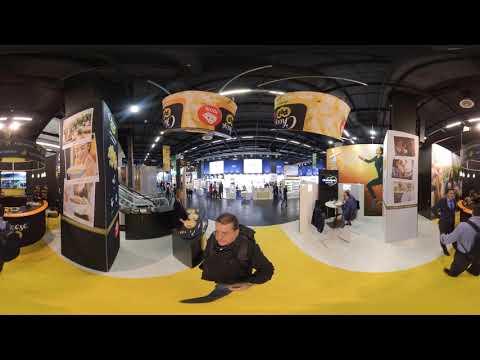The image depicts a bustling convention center with a yellow floor, segmented into numerous display stations. In the center, a Caucasian man with short brown hair, glasses, wearing blue jeans, a black jacket, and a backpack is holding what appears to be a 360-degree camera on a pole. The image presents a warped, panoramic view, likely resulting from a fisheye or 360-degree lens. To the right, another man in a lighter blue shirt, black pants, and a backpack converses with a man dressed in a dark suit with a blue shirt. Various white and black pillars are adorned with images, possibly depicting bowls of food, contributing to the decor of the temporary-looking booths. At the top of the image, large, sculpture-like constructions resembling giant ramen cups are visible, hinting at a possible food-themed exhibit. The scene leads into a brighter entryway, suggesting this could be a part of a larger trade show or an art studio setup.